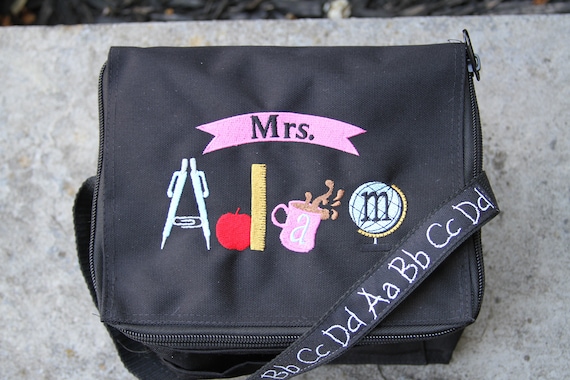This overhead photograph showcases a meticulously designed black nylon lunchbox, aimed at educators. The lunchbox, resting on a gray stone ledge, features a zippered top and an embroidered carrying strap with a repeating pattern of the alphabet in both uppercase and lowercase letters, resembling chalkboard writing. Prominently displayed on the top flap is a pink pennant-style banner with "Mrs." in bold black embroidery. Below the banner, the name "Adam" is creatively spelled out using classroom-themed items: two green pens angled to form an "A" with a paper clip, a red apple paired with a vertical yellow ruler for the "D," a pink coffee mug with spilling coffee for the second "A," and finally, a green globe representing the "M." This detailed and personalized design makes it clear that the lunchbox is tailored for a teacher named Mrs. Adam.